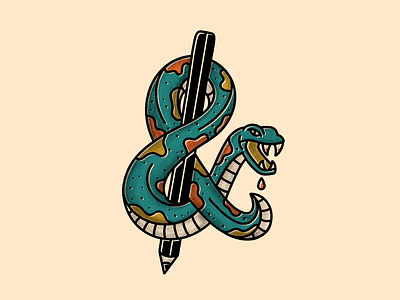In this high-quality cartoon image, a brightly colored snake is intricately wrapped around a vertically standing black pencil, which is pointed downwards. The scene is set against a light pink to tan background. The snake, which is primarily a vivid teal or turquoise color, features a combination of orange, yellow, and red irregular spots along its back. Its underbelly is white and segmented into small square shapes. The snake, coiled around the pencil in a figure-8 formation, has its mouth open displaying four sharp teeth, two on the top and two on the bottom. A teardrop shape near its mouth suggests venom dripping. The pencil, a traditional type that can be sharpened, stands out starkly against the soft background, emphasizing the coiled reptile's animated and vibrant design. There is no text in the image, allowing the focus to remain on the detailed depiction of the snake and pencil.